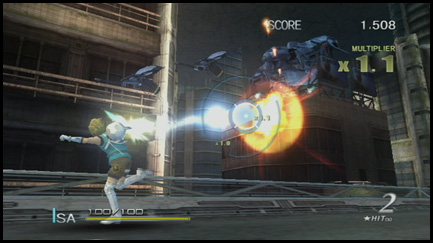This image depicts a gameplay screen, presented in a rectangular format. Positioned at the bottom left corner is a human-like character, distinguished by their prominent yellow head. The character's attire includes teal-colored topwear and black shorts, complemented by white shoes. On the screen, below the character, the text 'ISA' is visible. To the right of the character, the numbers '100-100' are displayed prominently. Further below, a yellow bar stretches horizontally across the screen. In the bottom right corner, the number '2' is featured, accompanied by artwork of a white star and the number '00' below it. This combination of elements suggests a detailed and structured gameplay interface.